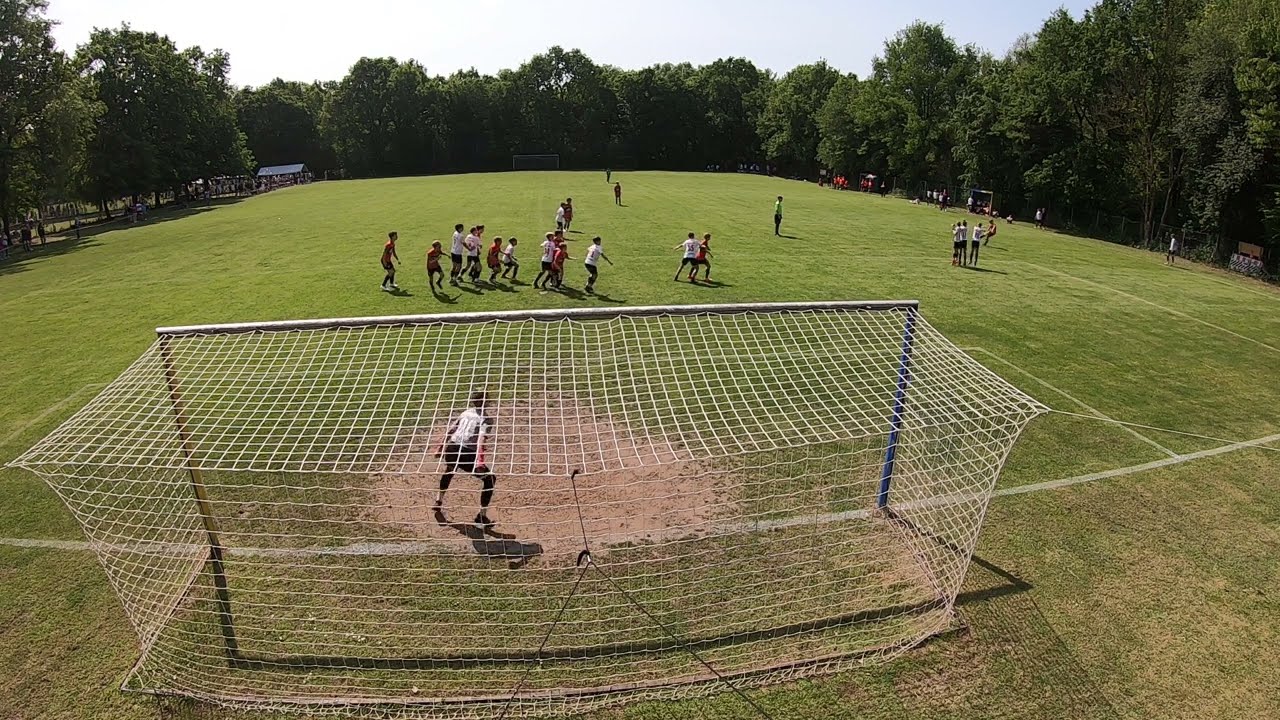The aerial view of the soccer field captures a vivid, dynamic scene. In the forefront, a prominent white net with a blue and silver frame stands out. Just in front of this net, a goalie is positioned with his back to the camera, dressed in a white or gray shirt and black leggings, seemingly poised for action. The shortcut grass of the field is meticulously marked with white lines delineating the various play areas and the edges of the field. Occupying the center of the field are players from two teams, identifiable by their red and black or white and black uniforms. The referee, distinguishable in a green jersey with black shorts, oversees the match. Around the edges of the field, spectators are seated in chairs, watching the game intently. Surrounding the entire field is a lush square of trees, their green leaves forming a natural, verdant barrier. Additionally, near the goalie's position, there are patches of dirt and mud, suggesting recent rain. This detailed scene encapsulates the energy and environment of a lively soccer match.